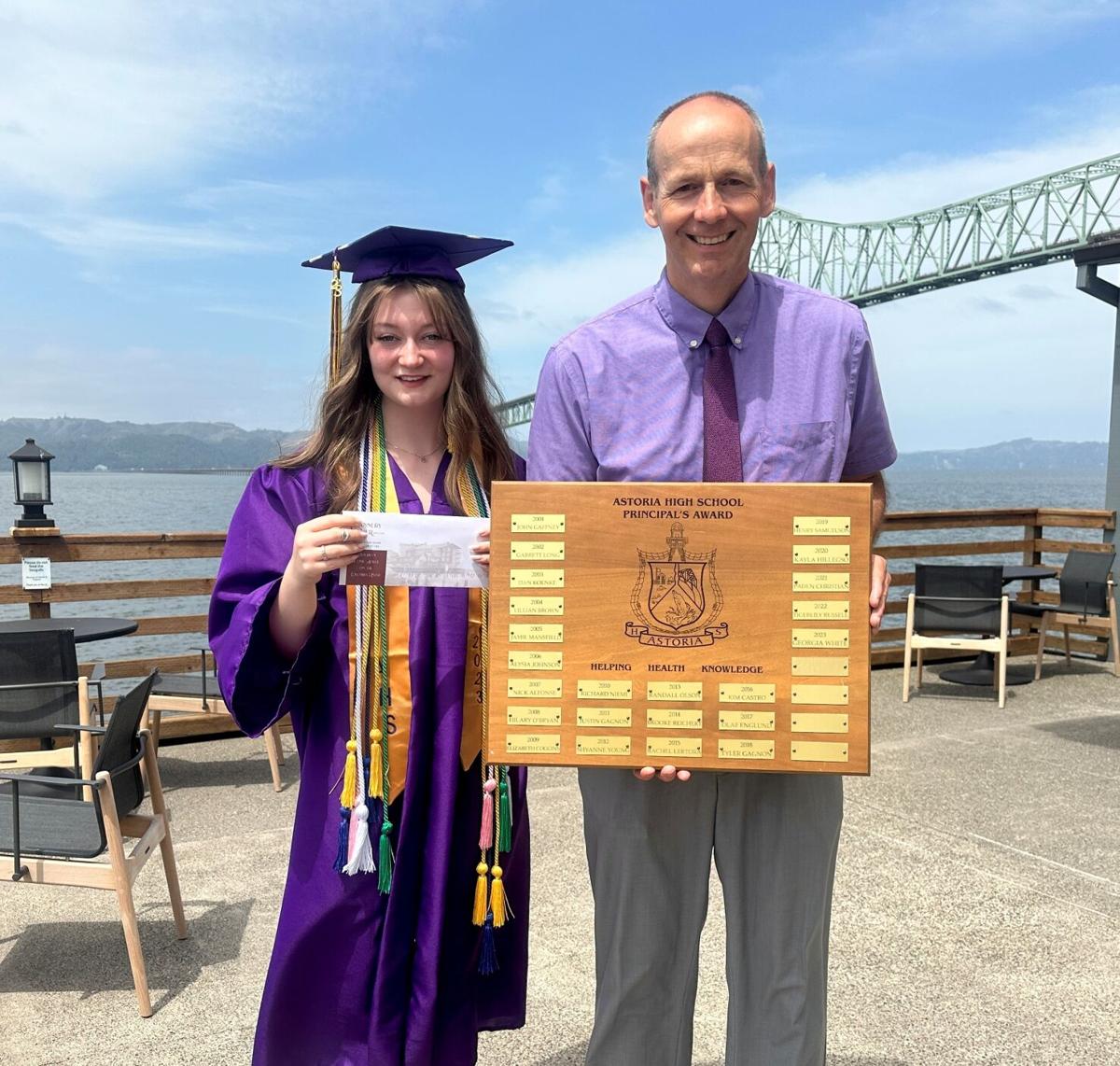In this vibrant outdoor photograph, set against a scenic backdrop, we witness a celebratory moment at a harbor area. Central to the image is a distinguished older man standing to the right, who appears to be either the principal or the father of the young woman on the left. The man, partially balding, is smartly dressed in a light purple collared shirt, a darker purple maroon tie, and gray dress pants. He holds a prestigious wooden plaque adorned with bronze nameplates and emblazoned with "Astoria High School Principal's Award" and the emblem of Astoria, showcasing a motto of "Helping, Health, Knowledge."

To his left stands a young woman, evidently a recent graduate, dressed in a bright purple graduation gown and matching mortarboard adorned with a green, yellow, pink, and white tassel hanging to her left. She has long, light-brown hair accentuated with blonde highlights cascading towards her thighs. Around her neck, she proudly wears multiple honor cords and an orange sash, signaling her outstanding achievements, though the text on the sash is obscured. She holds a rectangular piece of paper, possibly a certificate or award.

The picturesque setting includes a body of water stretching into the distance with a light green steel bridge partially visible, indicating a pedestrian or rail structure with distant hills or mountains beyond the riverbank. They stand on a light-colored pebble-dash concrete patio area featuring brown railings with a lamp atop, balsa wood chairs with black upholstery, and black circular tables, all under a bright blue sky with minimal clouds. The bridge and serene environment enhance the celebratory atmosphere of this proud graduation moment.